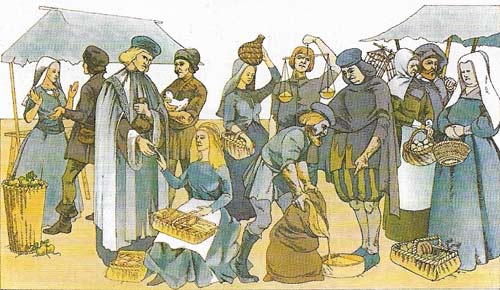The image is a panoramic, cartoon-style drawing depicting an old-era marketplace, likely from the biblical or medieval times. The foreground is bustling with roughly 12 to 15 men and women dressed in period-appropriate clothing such as tunics and pantaloons, engaging in various market activities. Central to the scene is a woman in a blue dress, seated with a basket on her lap, seemingly selling items. Surrounding her, a man to her left cradles a bird, while another to her right inspects a pair of handheld scales. Additional market activities include another man pouring grain from a sack into a pan, as a nearby individual points toward the transaction, and a woman carrying a basket of eggs. In the upper corners, two simple tents with peaked roofs created by wooden poles add to the marketplace atmosphere, augmenting the setting's historical and communal vibe.